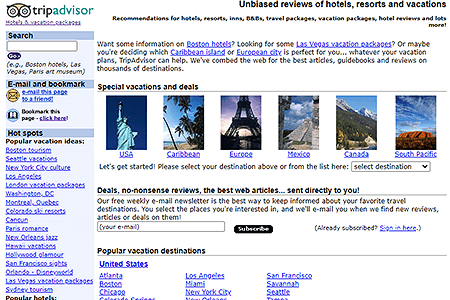The webpage on TripAdvisor features the familiar owl logo and the prominent heading "TripAdvisor." To the right, it states, "Unbiased reviews of hotels, resorts, and vacations." 

On the left-hand side of the page, there is a selection of destinations that users can choose from. Each option is accompanied by clickable text links for further information. Below this list, six clickable thumbnail images are displayed, each representing a popular travel destination: the USA with an image of the Statue of Liberty, the Caribbean depicted with palm trees, Europe with the Eiffel Tower, Mexico with what appears to be ziggurats in the jungle, Canada possibly showcasing the Rocky Mountains, and the South Pacific with an island scene.

The page also mentions features like "Deals," "No nonsense reviews," and "The best web articles sent directly to you," suggesting an invitation for users to subscribe to TripAdvisor for regular updates. The page itself appears to be a template in which no specific information has been filled in yet.